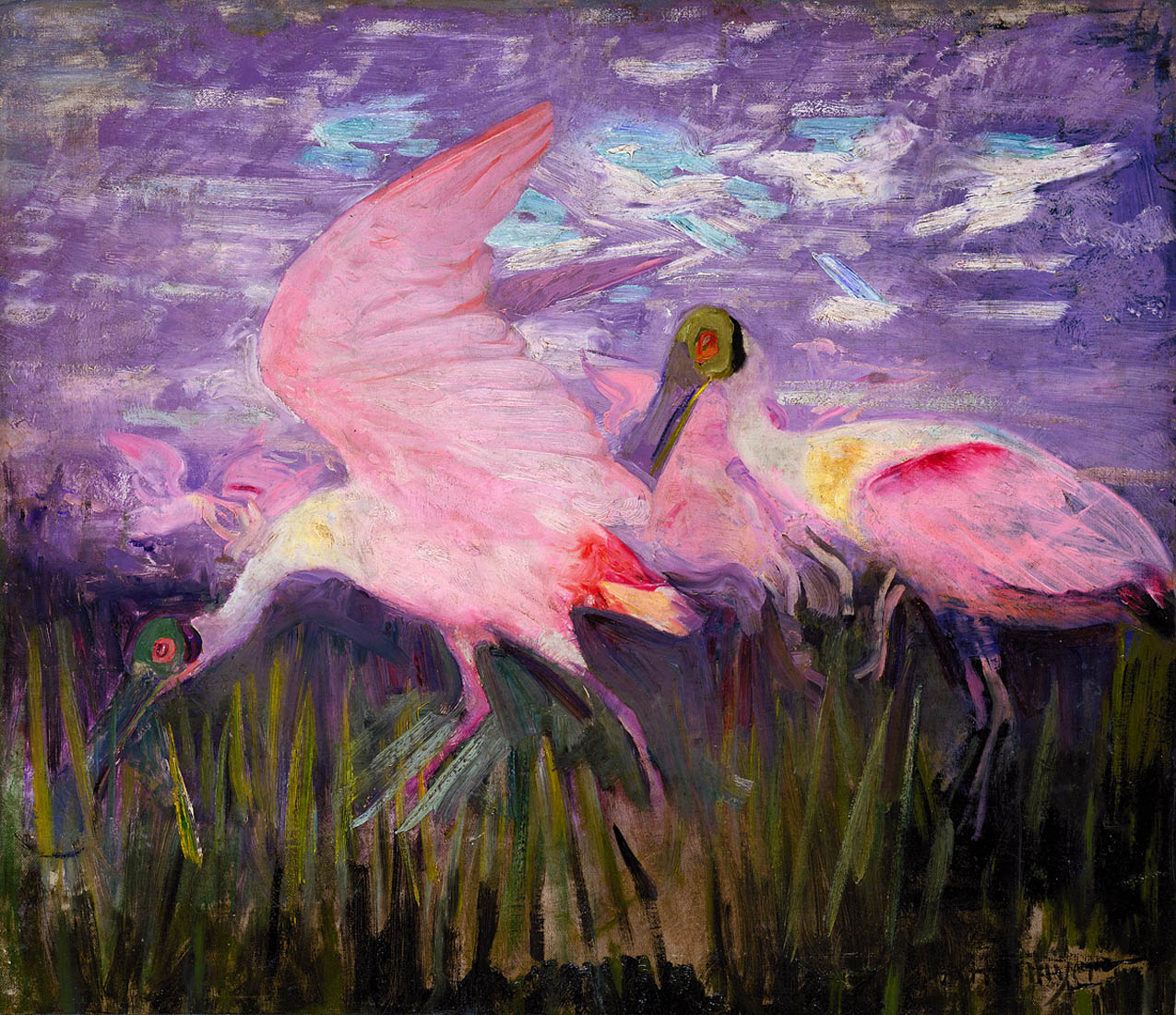The art piece beautifully displays a vibrant scene teeming with color, created using what appears to be acrylic paints applied with dry brush techniques, although some elements suggest possible watercolor or oil medium use. Dominating the scene are two fantastical bird-like creatures with strikingly detailed features and a rich color palette. Both birds possess bright green heads, with one having a blue beak and another a purple one, and their eyes are a vivid red. Their bodies consist of pinks and reds, with hints of orange, yellow, and muddled green tones. The surrounding environment is an abstract interpretation of a grassy pasture with reflective water-like qualities. The sky above is a harmonious blend of periwinkle purple, with brush strokes of light blue, white, and gray, along with abstract impressions of other birds flying. The image brims with various intricate brush strokes, particularly in the foreground bird’s open wings, conveying a dynamic sense of movement, as if ready to take flight.